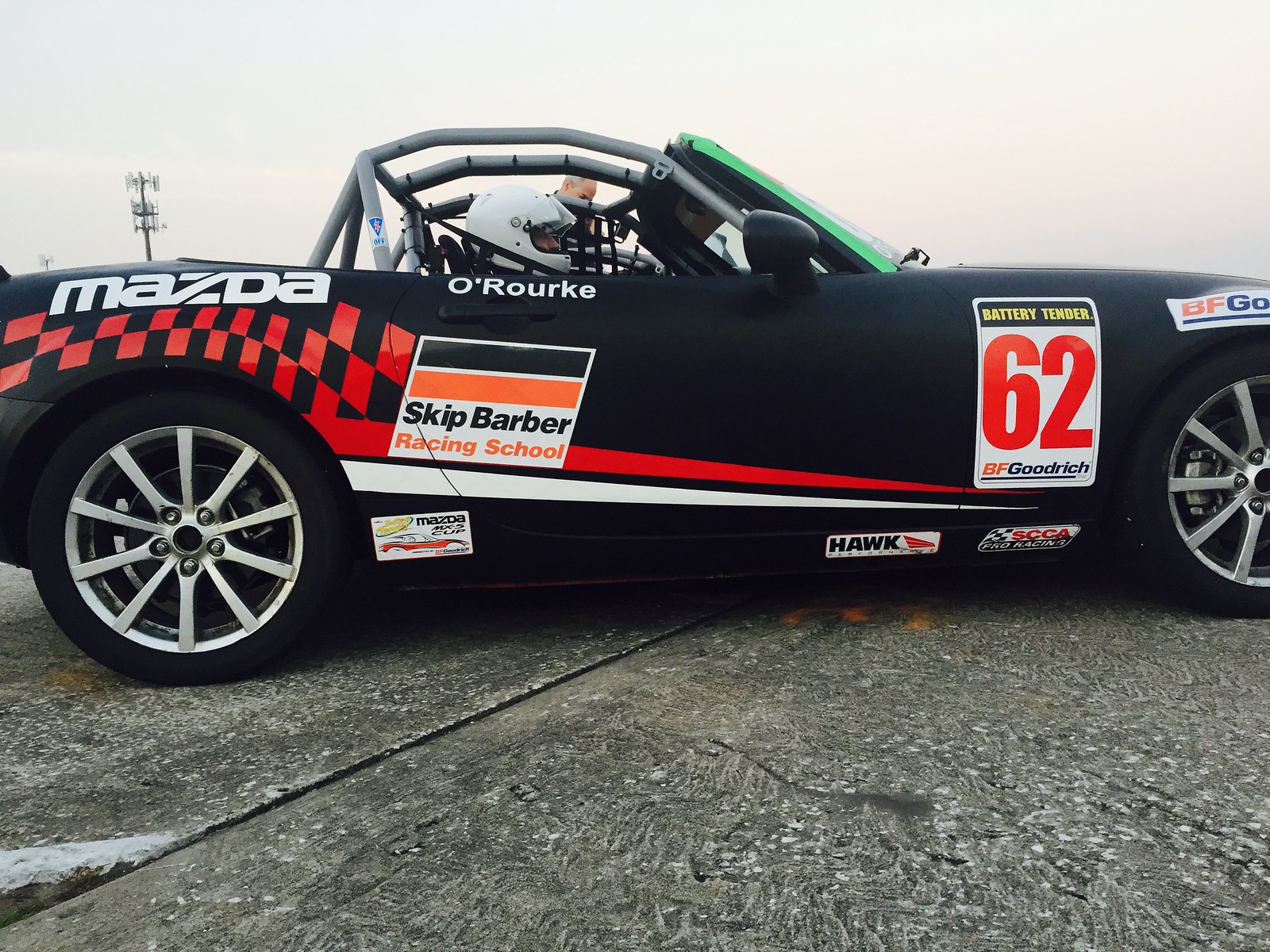The image depicts a sleek, black race car designed like a high-performance sports car rather than a stock car or an F1 vehicle. The car is adorned with a striking red and black checkered design on the rear panel near the rear wheel and features a prominent red stripe running down its side. Along the top left, the car displays the word "Mazda" in bold white letters. Just below that, on the driver's door, the name "O'Rourke" appears in white paint, indicating the driver’s name. Beneath O'Rourke's name, there is a red, orange, and white text box that reads "Skip Barber Racing School," signifying that the car might be part of a racing school fleet. Further along, a white box bears the number 62 in red. Above this number box, the logos "Battery Tender" and "BF Goodrich" can be seen.

The car is open on top like a convertible and equipped with a gray metal roll cage. The driver, wearing a white helmet, is visible behind the wheel. Near the rear of the vehicle, an older gentleman stands outside the car. The scene is set on a gray, concrete pavement under what appears to be an overcast sky, adding a dramatic background to the image. In the distance, a telephone pole with large lights is faintly visible, emphasizing the car's presence on a race track.